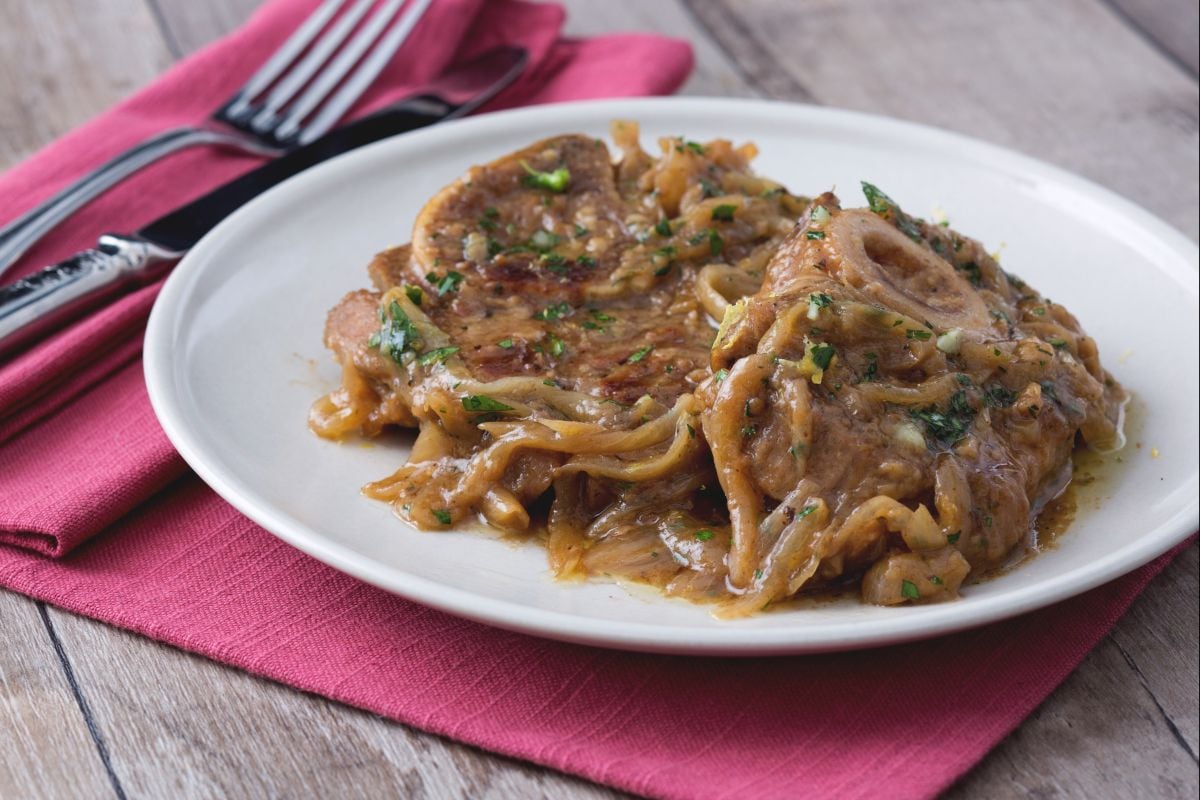The image showcases a meticulously presented meat dish, likely a pork chop or pot roast, garnished with fresh cilantro and possibly chives. The succulent cut of meat is bathed in a rich, thick gravy, with visible onions on the edges, suggesting a deeply flavorful preparation. Resting on a clean, minimalistic white plate, the dish is complemented by the natural textures of a maroon tablecloth underneath it. Accompanying the plate are a silver knife and fork placed to the left, creating a balanced composition. The setting is further enhanced by an ash-gray wooden table that spreads beyond the frame, providing a rustic backdrop. The excellent lighting and high image quality suggest a professional photo shoot, potentially capturing the dish in stunning, natural outdoor light.